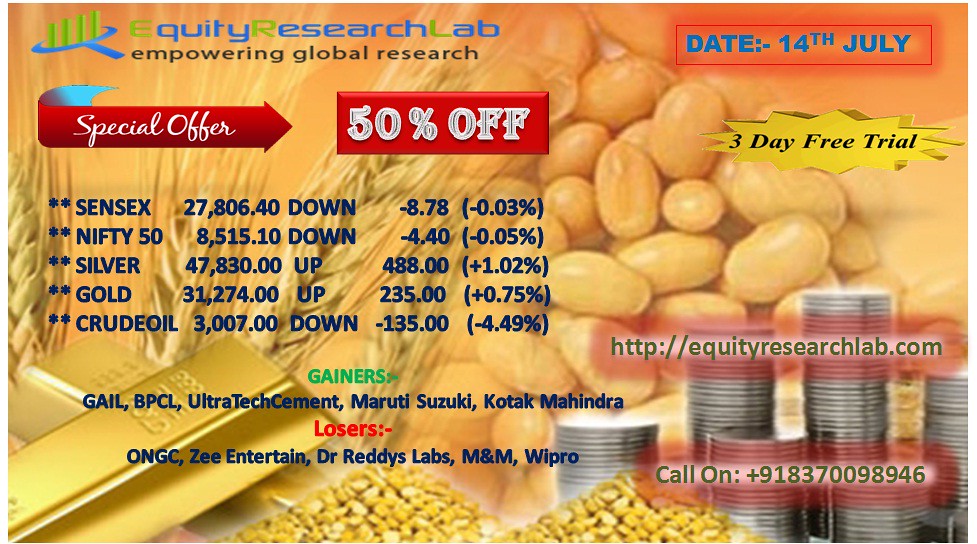This detailed caption describes a screenshot of a website with a focus on market research and commodities trading:

---

The screenshot showcases the homepage of "Equity Research Lab," a website dedicated to empowering global research. In the upper left-hand corner, the site’s logo and tagline, "Equity Research Lab: Empowering Global Research," are prominently displayed. The upper right-hand corner shows the date, "14th July," along with a marketing prompt for a "Three-Day Free Trial."

Centrally located on the page is a vibrant banner highlighting a "Special Offer: 15 or 50% Off." Beneath this offer, there is a detailed list of various commodities and indices, including Sensex, Nifty Fifty, Silver, Gold, and Crude Oil, each showing their current trends—whether they are up or down—and the specific value changes associated with them.

Further down, the page is divided into two sections: "Gainers" and "Losers," which enumerate companies that have experienced notable gains and losses, respectively.

The background image includes visuals that evoke a real-world connection to commodities, featuring close-up photographs of corn kernels and stacks of silver coins.

---

This caption thoroughly details the elements present on the webpage, capturing the layout, informational content, and the thematic imagery used in the background.